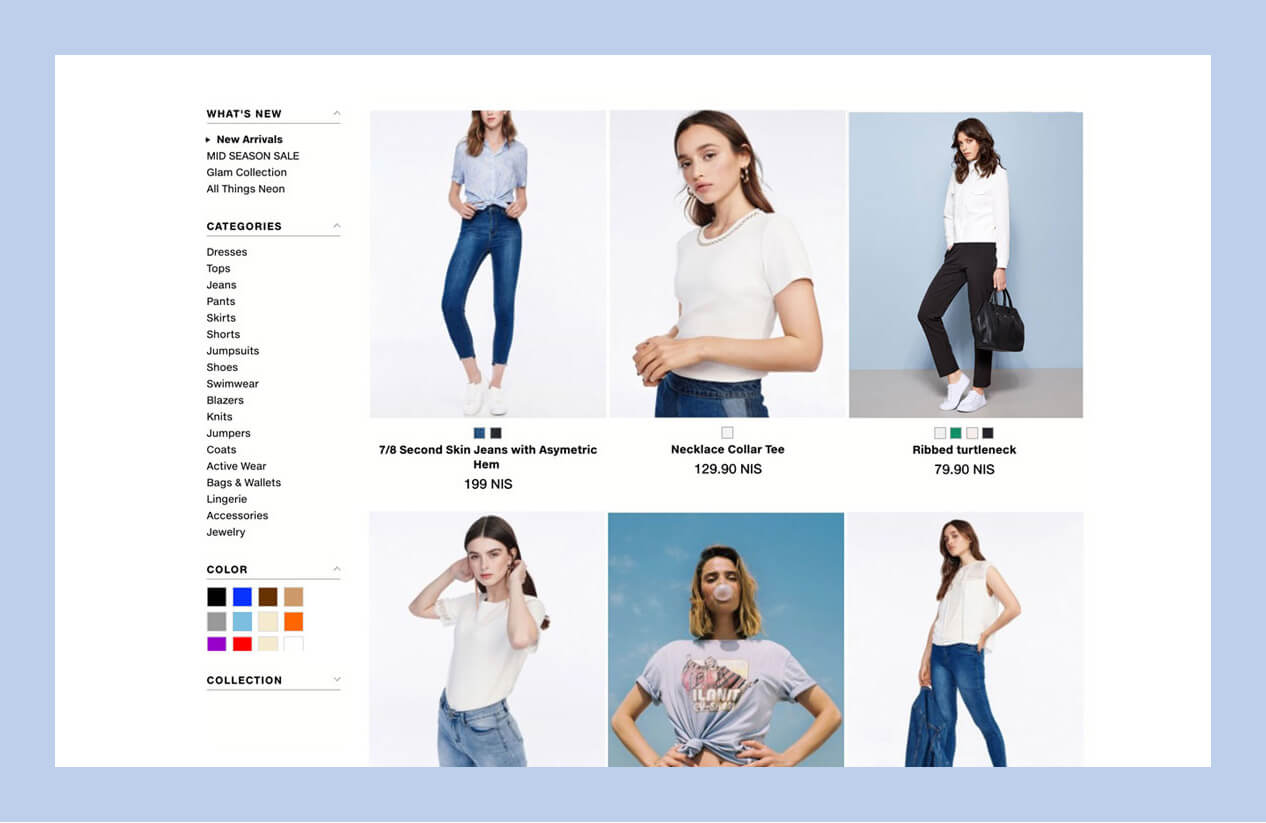The webpage of a women's clothing site showcases six models, all Caucasian women with similar features but not identical. They are dressed mostly in trendy summer attire, with light-colored, short-sleeved tops and some in jeans. Among the six images, one model stands out in a ribbed turtleneck, giving off a slightly wintry vibe, and she is carrying a bag in her left hand. The left sidebar features various shopping categories including dresses, tops, jeans, pants, skirts, shorts, jumpsuits, shoes, swimwear, blazers, knits, jumpers, coats, activewear, bags and wallets, lingerie, accessories, and jewelry. There are options to filter items by color and tabs for new arrivals, a mid-season sale, and a glam collection, with new arrivals currently selected. Prices are listed in NIS (New Israeli Shekel), such as the ribbed turtleneck priced at 79.90 NIS.